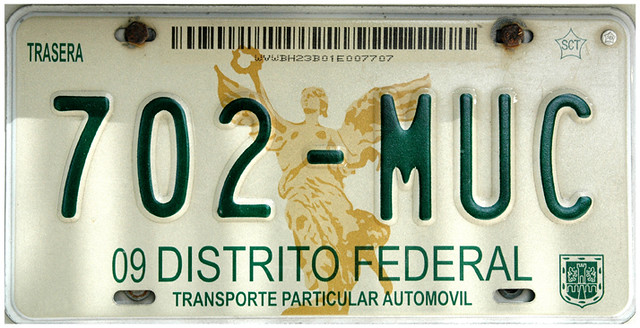The image features a Mexican license plate, distinguished by its white background and numerous detailed elements. At the center of the top edge, a large black barcode is prominently displayed. Directly beneath the barcode are the numbers "WVWPH23P01A007707" in black text. To the left in green text is "TRASERA." The license plate number "702-MUC" is centrally positioned. Below this, the inscription "09 Distrito Federal" followed by "Transporte Particular Automobile" is visible. 

A bronze-colored emblem of an angel, characterized by wings and a raised hand, decorates the center of the plate. Rusty screws secure the license plate at the top left and right corners. On the top right is a green star logo with "SCT" written in green letters. The bottom right corner features another green logo, the specifics of which remain unclear.